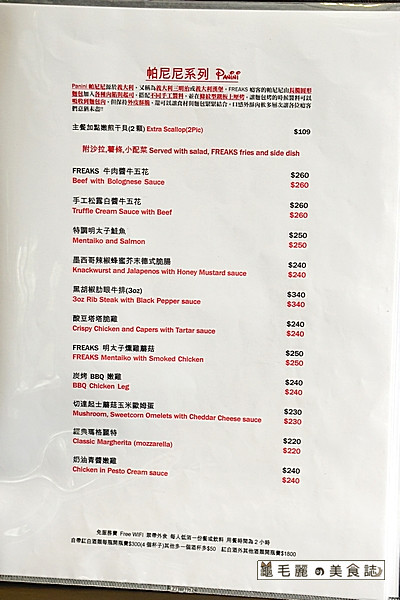The image depicts a detailed menu printed on white paper, predominantly featuring Asian text interspersed with English descriptions. At the top center, some items are highlighted in red and underlined, with "Panini" mentioned next to these items.

Proceeding downwards, in red text, "Extra Scallop, $100" is prominently displayed. Below this, there is the phrase, "Served with salad, freak fries, and side dish." Listed in black is "Freaks, $2.60." Following this, in red lettering, "Beef with Bolognese Sauce, $2.60" is specified, accompanied by more Asian writing with the same price.

Further down, "Truffle Cream Sauce with Beef" is listed at $2.60 in red, followed by more Asian text priced at $250. Next, "Mitako and Salmon" appears, priced at $2.50. More Asian text, priced at $2.40, follows. "Knackwurst and Jalapenos with Honey Mustard Sauce" is featured next at $2.40, followed by Asian text priced at $3.40. 

"3 oz Rib Steak with Black Pepper Sauce" and "Crispy Chicken with Capers with Tartar Sauce" are listed next, at $3.40 and $2.40 respectively. In red text once again, "Freaks and Taco with Smoked Chicken, $2.50" appears, followed by "Barbecued Chicken Leg" in red for $2.40. "Mushrooms, Sweet Corn Omelets with Cheddar Cheese Sauce" is listed at $2.30, accompanied by Asian text, then "Classic, Margarita, Mozzarella, $2.20."

Towards the bottom, more Asian writing is visible, along with "Chicken and Pesto Cream Sauce, $2.40." The entire menu is cleanly presented on what appears to be a standard piece of white paper.